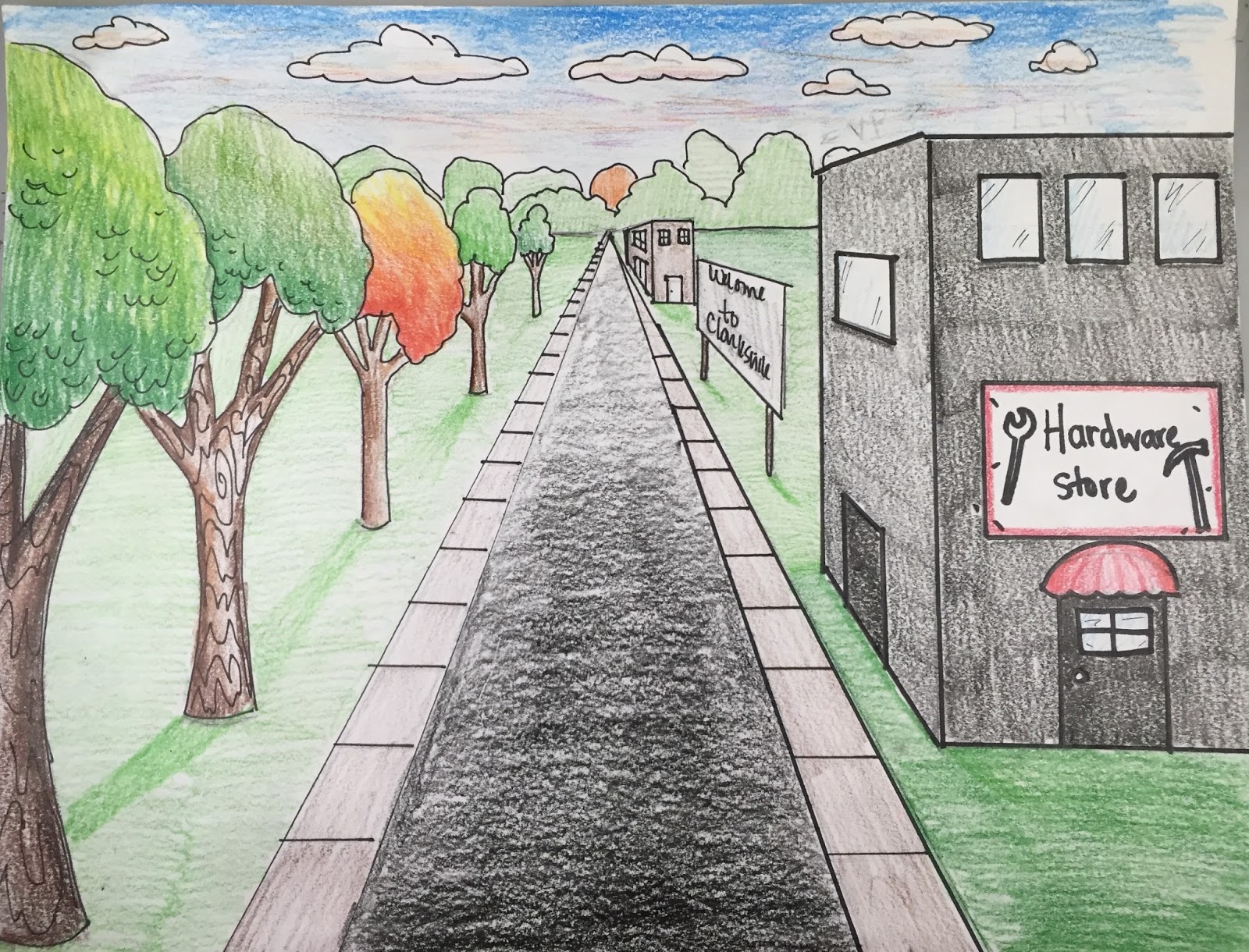This drawing, likely created by a teenager, showcases a vivid depiction of a city street extending into the horizon. Rendered in crayon, the artwork features vibrant elements: a black street in the middle flanked by gray sidewalks with defined lines, lush green grass, and a variety of trees, including green, brown, and orange ones, especially pronounced on the left side. The sky above is a striking blue with white clouds and hints of purple, complemented by an orange sun setting behind the bushy trees in the background.

On the right side of the drawing stands a detailed, two-story gray building identified as a hardware store, complete with a white sign, pink awning, windows, and a black door. Adjacent to the store is a "Welcome to Clarksville" sign, adding a touch of locality to the scene, followed by another building further in the background. The combination of these elements with the crayon's rich texture and childlike charm, enhanced by skilled use of perspective and angles, creates an engaging and detailed urban landscape.